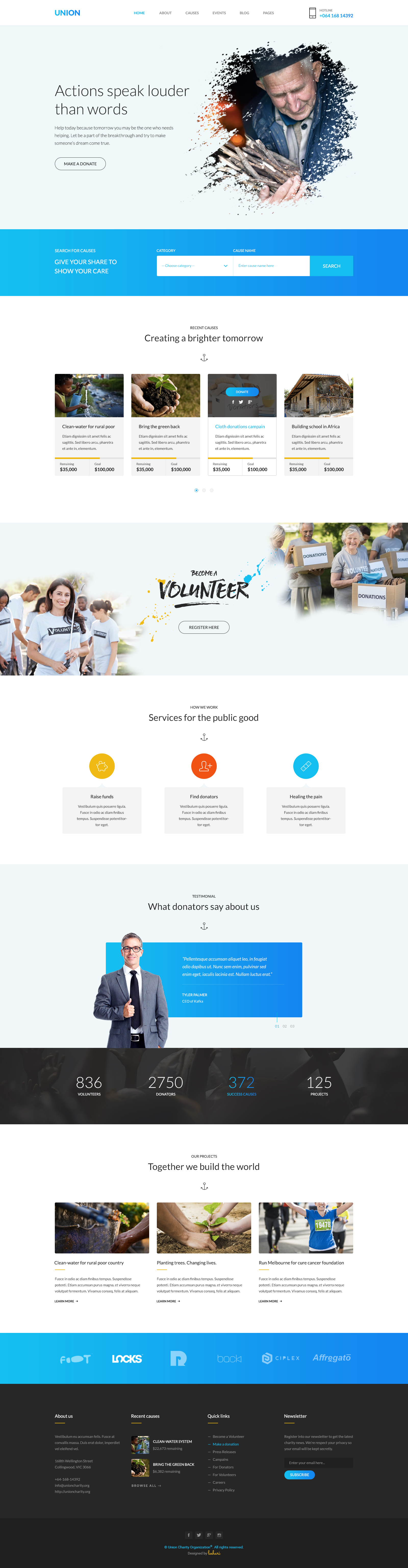The image depicts a website with the headline "Actions Speak Louder Than Words" prominently displayed at the top. Below the headline, there is a photograph of an older man dressed in a suit and a white button-down shirt, looking downwards while holding what appear to be sticks. 

At the bottom of the website is a blue bar, within which lies a white search bar accented with blue at the end. Below this section are four distinct images: one of hands holding dirt, one of a house, one that features a simple blue bar, and another that is less discernible, showing something white with a hint of blue.

Further down, there is a box containing text about volunteering, accompanied by an image on the left side of people in white t-shirts engaging in activities. In the upper left of this section, older individuals are seen carrying boxes. There are three circles in gold, red, and blue below this part.

Underneath, there is a statement with a picture of a man in a suit and tie in front of a blue background. A black strip featuring numbers or images runs across this area. Below this strip are three more image boxes, and further down, there is a box with a blue header and black base, containing information too small to be legible.